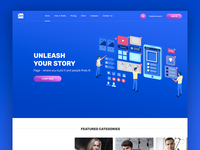A visually overwhelming webpage features a predominant bright blue color scheme. The main background is a vibrant blue, with a slightly different shade of blue used for a central rectangle. Atop this central rectangle, in bold, white text, is the readable headline: "Unleash Your Story." Directly beneath this, smaller white text is present but illegible due to the poor resolution. A red button also appears within this area, though its inscription remains unreadable. 

The page's navigation bar, located at the top, comprises white text links that also suffer from poor legibility. Additional red buttons, including a round one and an oblong one, are present along with a potentially blue button – all of which share the unreadable text issue.

The visual content includes an image of a cartoon figure – possibly a representation of the same man repeated three times. This character is dressed in blue jeans and a yellow t-shirt, depicted in the process of working on something attached to a wall. Below this illustration is a white text area bearing black text, though it is cut off and also unreadable.

Towards the bottom of the page, three small photographs show individuals' heads, but the accompanying text is too blurry to decipher even when viewed at a larger size. In essence, apart from the prominent "Unleash Your Story" message, the webpage suffers from a lack of clarity and legibility across its various elements.